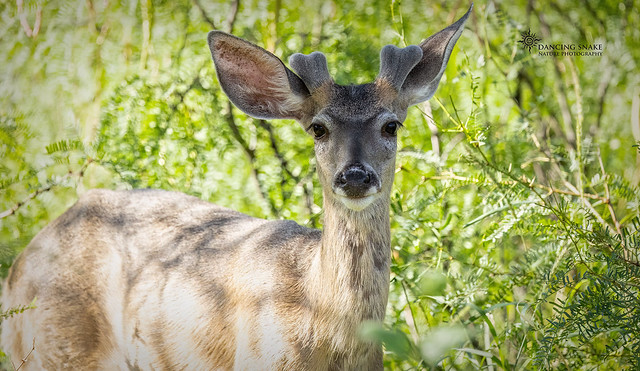The photograph features a young, light tan female deer standing in a woodland area, captured in a professional and serene setting. The deer, characterized by its large, pointed ears, stands out as it gazes directly at the photographer with a calm and inquisitive expression, possibly having just paused from grazing. The natural lighting gently illuminates the deer's face while shadows from the surrounding foliage add depth to the scene. In the upper right corner, a watermark with the text "Dancing Snake Nature Photography" and a circular star or sun logo subtly marks the image. The background showcases a lush, forested area with greens interspersed with light browns, further framing the tranquil portrait of the deer.